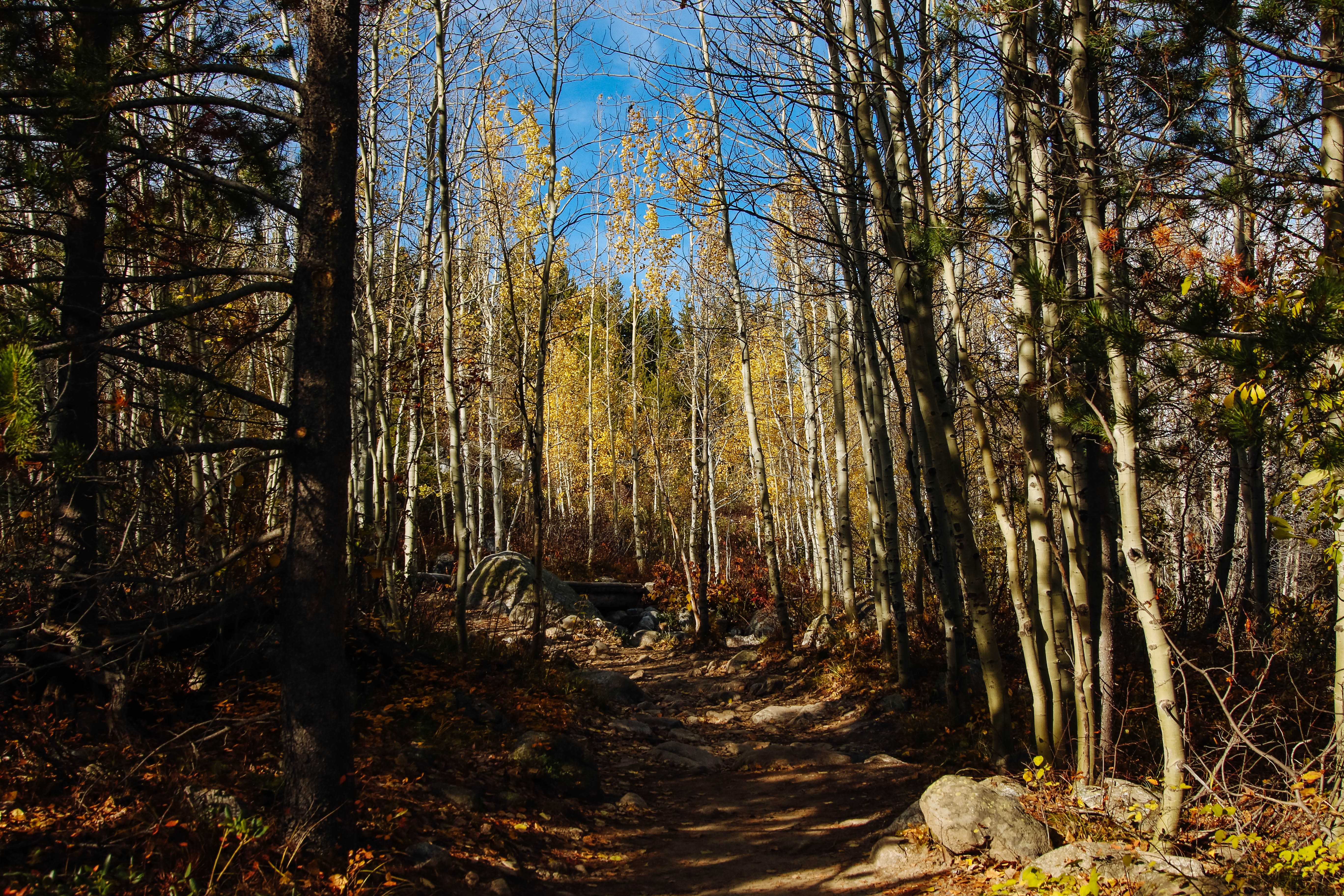This is a detailed photo taken in a wooded area, featuring a dirt walking trail winding through the forest. The area appears to be a mix of tall, lanky trees, mostly bare, indicative of late fall or early winter. These trees are primarily bare with a few holding onto their brownish-green and dark green pine needles. The light filters through the canopy, casting a mix of light brown and black shadows across the landscape. The trail itself is lined with gray rocks and small to medium-sized boulders, and vibrant green patches can be seen on the forest floor, especially toward the bottom right corner. In the distance, more trees with yellow leaves can be seen, adding a touch of color to the scene. A notable feature is a large boulder on the right side, around which the trail curves. Adjacent to this boulder, there is a fallen log crossing a small ditch. The blue sky overhead indicates that the photo was taken during the daytime.